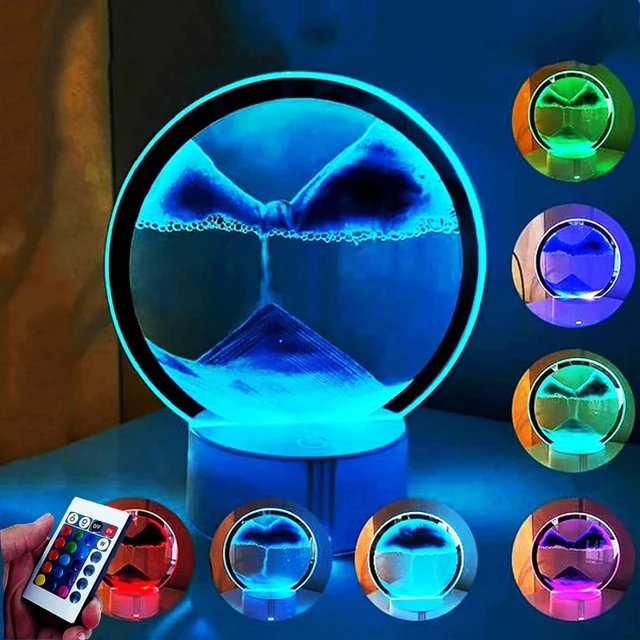The image depicts an advertisement for an LED light product, prominently featuring a central, larger LED light with a liquid-like interior that illuminates in various colors. This main light, outlined in black and emitting shades of blue, is the focal point of the image. Surrounding this primary light, there are eight smaller circular LED lights placed at the bottom of the image, showcasing a spectrum of colors including red, different shades of blue, green, and purple, akin to miniature lava lamps.

In the bottom left corner, a hand is seen holding a remote control, which is designed to adjust the colors and power of the LED lights. The remote features distinct white buttons for turning the lights on and off, along with multiple buttons for color adjustments, including a top button marked with a ‘W’ likely indicating white light. The background of the image is predominantly dark blue with a blue platform where the products rest, offset by a section of dark brown to the left.

No text is present in the image, emphasizing the visually striking display of the vibrant LED lights, further enhanced by the good quality of the photograph.